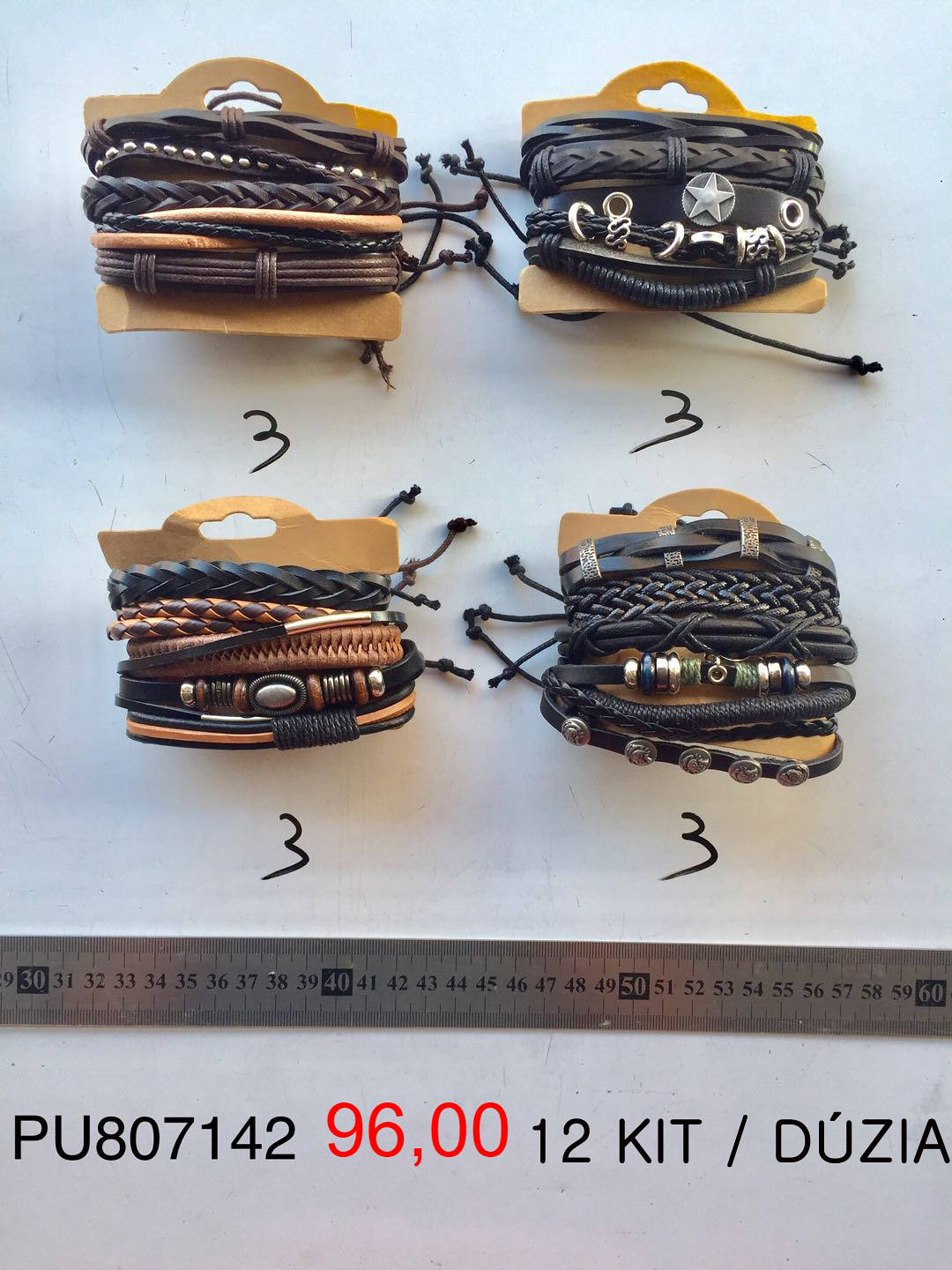The image depicts four sets of leather bracelets wrapped around cardboard sections. Each set has a handwritten number “3” in magic marker beneath it. A silver metallic ruler measuring their length stretches horizontally across the bottom of the picture, displaying the measurements against a white background. Below the ruler, there's black text reading "PU 807142," and red text stating "96,00." Additionally, black text spells out "12KIT-DÚZIA," suggesting a different language. The bracelets, varying in shades of brown and gray, feature intricate woven designs and include attached charms such as stars and buckles. These items appear intended for display or sale, possibly in an online store.